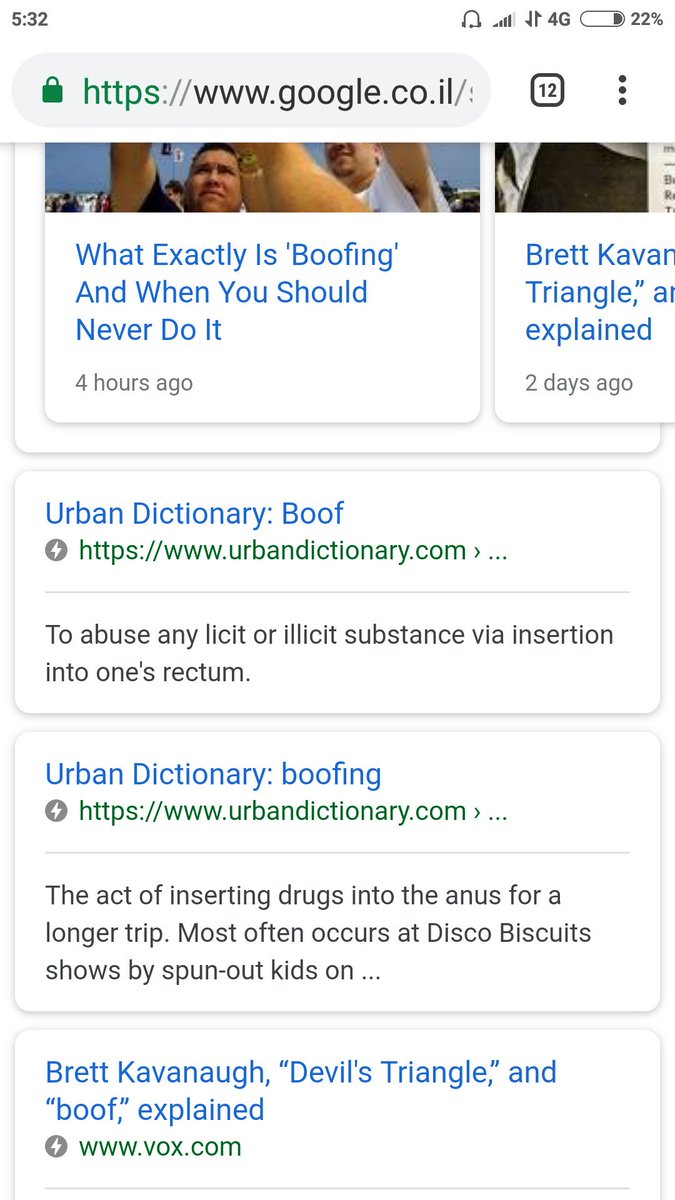This image captures a screenshot taken in portrait mode on a smartphone. In the upper left-hand corner, the time displays as "5:32". The battery level shown in the upper right-hand corner is at 22%. Below this, there is a search bar showing the URL "google.co.il" along with an icon indicating that there are 12 open tabs, and a menu symbolized by three vertical dots. 

As the user scrolls down the page, only the top portion of an image featuring two men is partially visible, accompanied by another image on the right. Underneath this, there is a blue, clickable link titled "What exactly is boofing and when should you never do it," which was posted four hours ago. Adjacent to it, text reads "Brett Cavan triangle explained," indicating content published two days ago.

Further down, the definition from Urban Dictionary is shown: "Boof: to abuse an illicit or illicit substance via insertion into one's rectum," with a green link directing to UrbanDictionary.com. Reiterating the theme, another entry from Urban Dictionary defines "boofing" with the same link, and elaborates: "The art of inserting drugs into the anus for a longer trip most often occurs at disco biscuits shows by spun out kids. How horrible."

The final section covers "Brett Cavanaugh Devil's Triangle and boof explained" with a green link to vox.com.